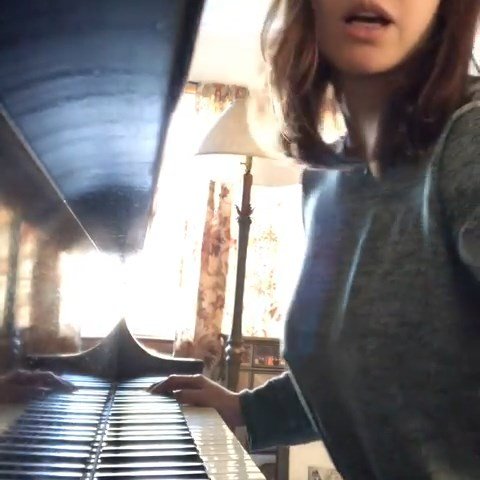This detailed photograph captures a young woman, her identity partially obscured as only the lower part of her face is visible, sitting at an upright piano in a cozy living room. Her shoulder-length brown hair frames her face, and she is clad in a gray long-sleeved shirt. Her right hand rests gently on the piano keys as if poised to play or in mid-performance. The setting includes floral curtains and a wooden standing lamp ornately carved with leaf patterns, adding a touch of vintage charm to the room. To her side, a picture rests on the floor, and a coffee table is discernible in the background. The piano, notable for its black and white keys, dominates the left side of the image while the woman occupies the right. The composition of the photograph is a vertical rectangle, offering a nearly square close-up view that emphasizes the intimate and homely atmosphere of the scene.